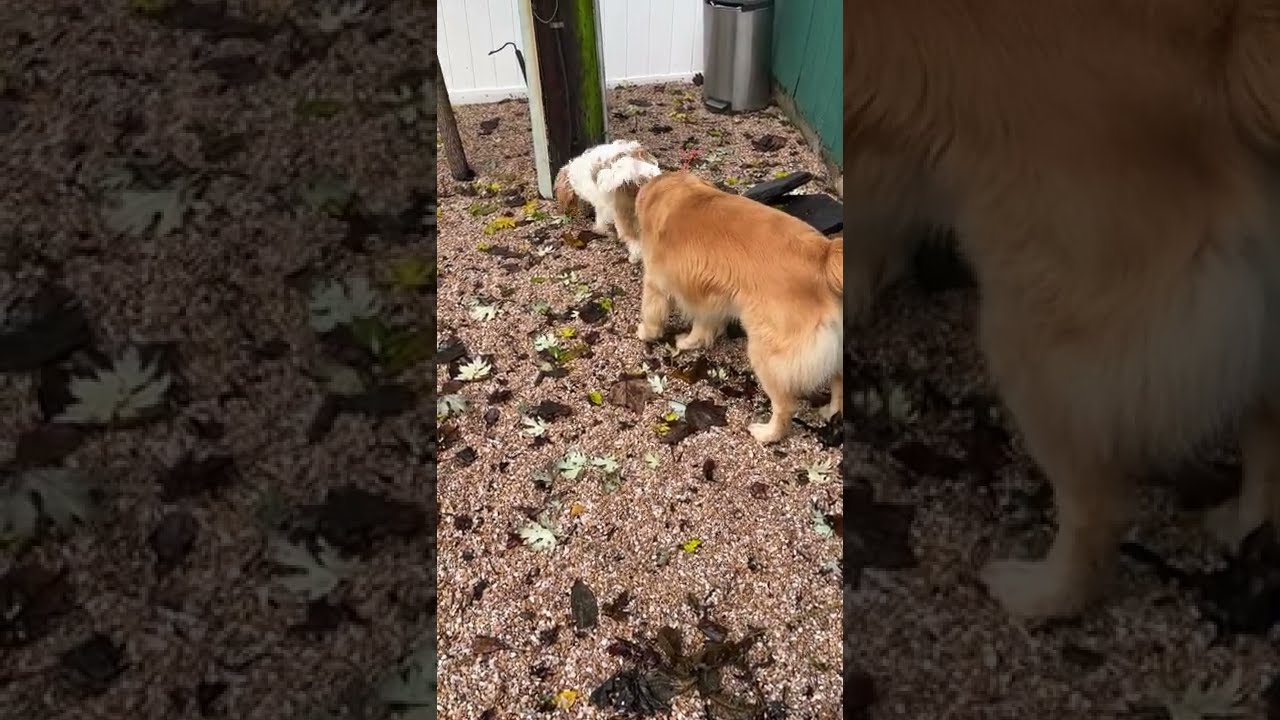This photograph captures two dogs standing on a ground covered in tiny gravel and scattered leaves, both green and dried. The dogs are positioned one behind the other, with the larger one at the back. The larger dog has orangish-brown fur with patches of white, while the smaller dog in front has white fur adorned with a beige stripe and floppy ears, seemingly drinking something. The setting appears to resemble a backyard, bordered by a white wall in front and a green wall to the right. In the background, there is a silver cylindrical trash can with a foot pedal, situated in the far corner. Additional details include a couple of poles and what appears to be a tree trunk in the upper left of the image, as well as some unidentifiable black objects nearby. Overall, the scene depicts a tranquil moment of the dogs exploring or searching for something amidst the gravel and leafy ground.